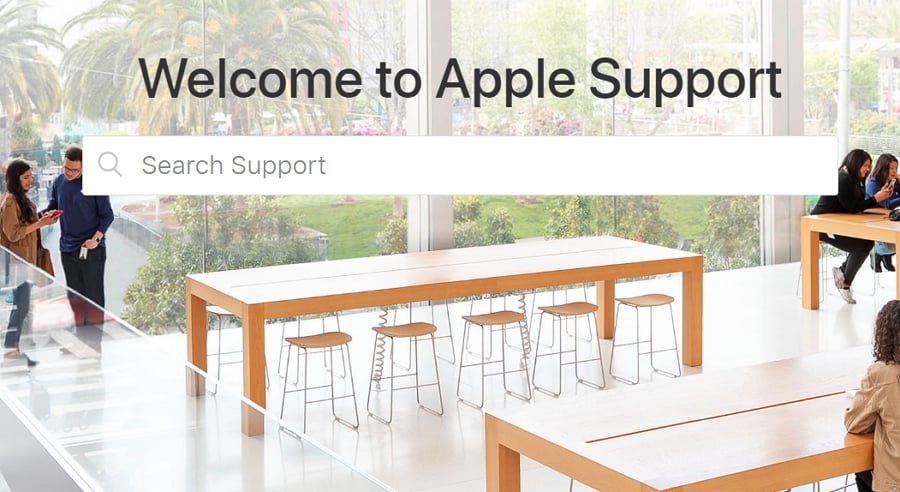The image captures the welcoming page of Apple Support, prominently displaying the phrase "Welcome to Apple Support" in bold black letters. Below this greeting lies a search bar labeled "Search Support," inviting users to find assistance. 

In the depicted setting, a spacious and contemporary area features several wooden tables, varying in width and featuring central slots—possibly intended for partitions. The table directly beneath "Search Support" remains unoccupied, surrounded by modern, sleek stools that might concern parents with young children due to their design.

To the right, another table accommodates seated individuals engaged in activities. Further in the background, a wider table hosts more people, with some engaged in conversation on the left side. The overall ambiance suggests a possible lunchroom setting.

The area is characterized by glass walls adorned with white square pillars, allowing an abundance of natural light to flood the space. Lush tropical plants can be seen outside, adding to the airy and open atmosphere. The choice of such an environment for the Apple Support page might not directly evoke feelings of support but instead highlights modernity and openness.